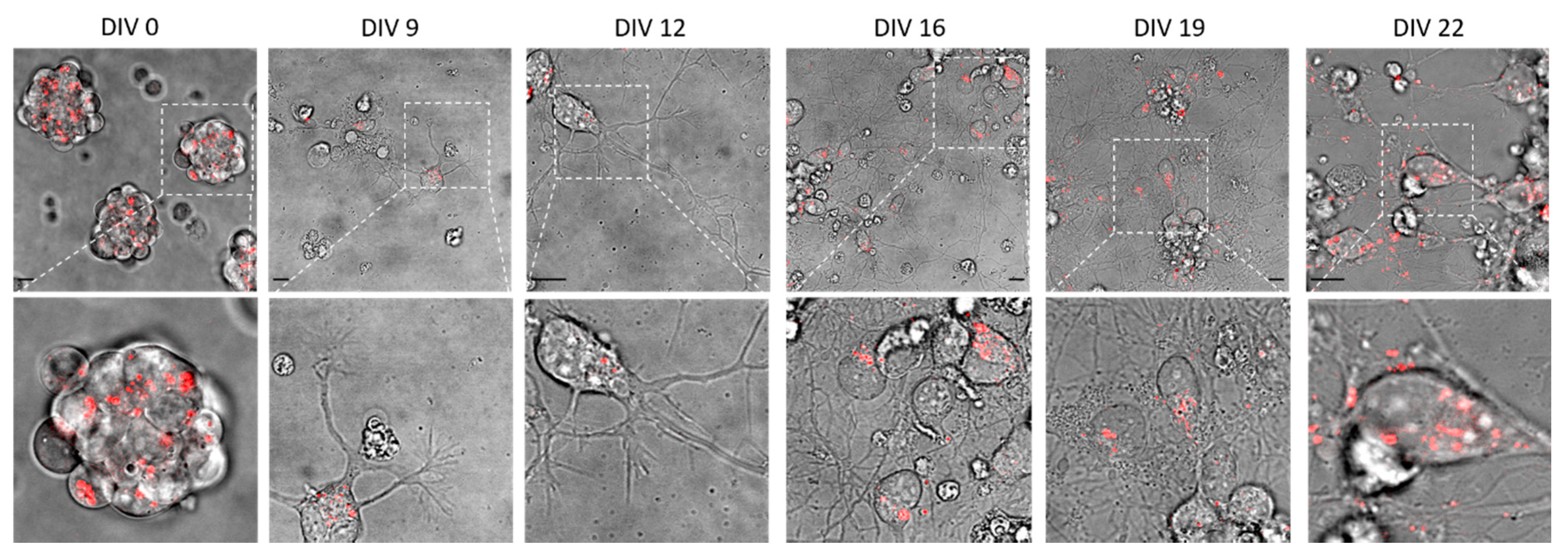The image appears to be a detailed diagram from a biology class, illustrating the growth and expansion of cell clusters over time. The diagram contains a total of 12 images arranged in two sets of six blocks. Each set corresponds to different time points of cell division, labeled as DIV0, DIV9, DIV12, DIV16, DIV19, and DIV22. The first image in each set provides an overview, while the second image is a magnified view of a specific area highlighted with a dotted line in the corresponding overview image. The clusters of cells are typically gray with some black outlines, and certain areas show prominent red clusters. These images depict various stages of cell or organism growth as observed under a microscope.